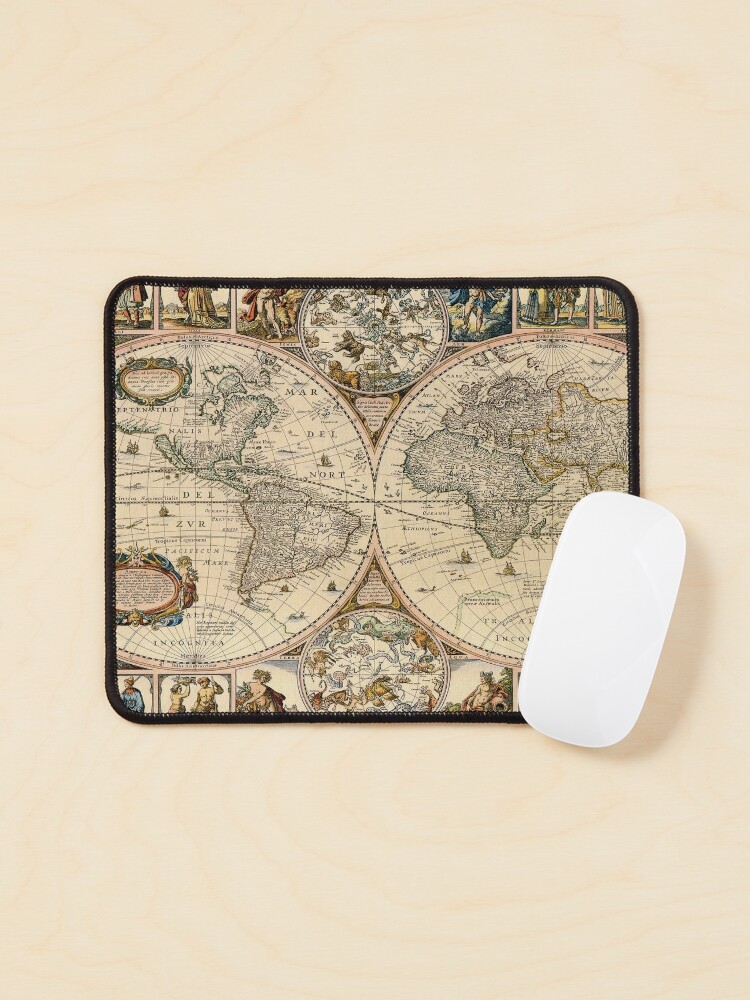This advertisement showcases a computer mouse pad designed with an old-timey world map. The mouse pad features intricate details in muted sepias, browns, pale blues, yellows, and oranges, all set against a cream-colored, marble-like background with slightly darker marbling. The map is neatly framed with a brown stitched edge, giving it a vintage feel. Surrounding the map are faded Renaissance-style paintings of Greek and Roman mythological figures, though they are partially cut off. The map displays detailed diagrams of the Earth’s landmasses, including continents such as Africa, Europe, and the Americas, arranged on two hemispheres with visible longitudes and latitudes. A white, sleek, wireless computer mouse, resembling an Apple mouse, is positioned at a 45-degree angle in the bottom right corner, just touching the mouse pad, adding a modern touch to the otherwise historical design.